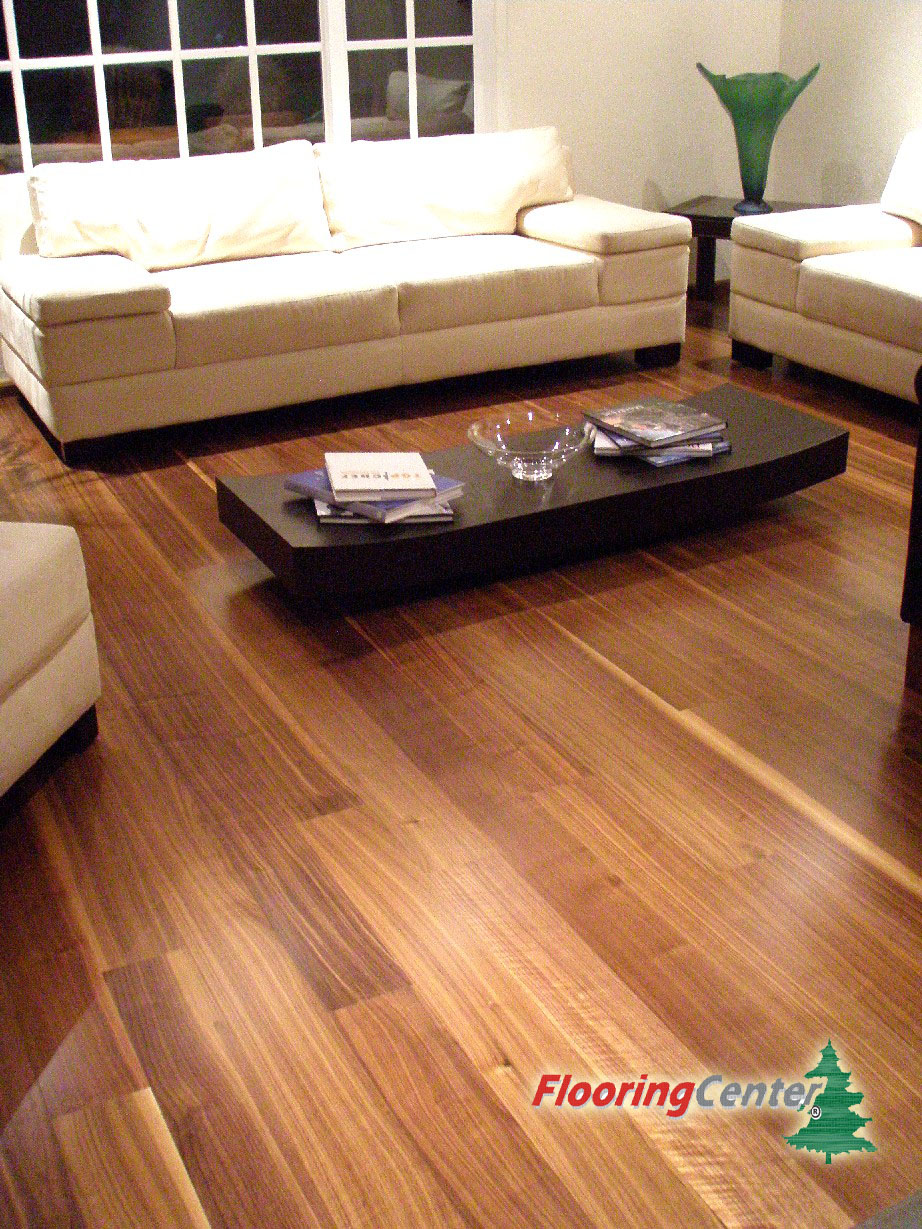The image is an advertisement for a flooring company, prominently featuring the text "Flooring Center" in the bottom right corner, with a small pine tree logo next to it. The flooring showcased is a lighter shade of hardwood, possibly a maple, that extends across a spacious living room. The room is decorated with white walls and a large, segmented window behind a white sofa, indicating it's nighttime outside. 

In the center of the room, there is a short, rectangular dark brown coffee table. The table holds a glass bowl in the middle and several books on either side of it, arranged in slightly tilted stacks of three or four. A white loveseat is positioned to the right of the window, and there's a white sofa in the background under the window. 

Additionally, in the back right corner, there’s a brown end table with a green vase, shaped almost like a V, placed on it. These elements all contribute to an inviting, contemporary living room setting that highlights the beauty and elegance of the lighter hardwood flooring.